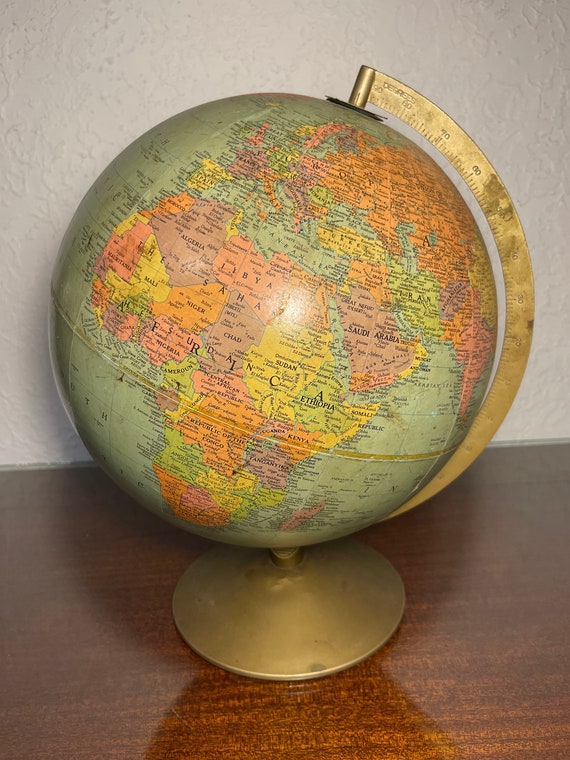This detailed image shows a side view of a vintage globe prominently featuring the continent of Africa. The globe stands on a tarnished, weathered bronze-colored base with a matching semicircular arm that wraps from top to bottom on the right side, featuring intricate numbering. The oceans are depicted in a faded blue, while the various countries within Africa and beyond are illustrated in subdued hues of yellow, orange, green, and pink, reflecting the globe’s age. The globe has a slightly tilted orientation, adding to its classic appearance reminiscent of those found in old schoolrooms. Resting on a glossy, deep brown wooden table, which may have a cherry undertone, the globe casts a faint shadow. The table itself is positioned against a textured white or light gray stucco wall with a pattern of lines. The globe's surface shows signs of aging with several scratches and brown stains. Overall, this image captures the essence of a timeworn yet educational artifact.